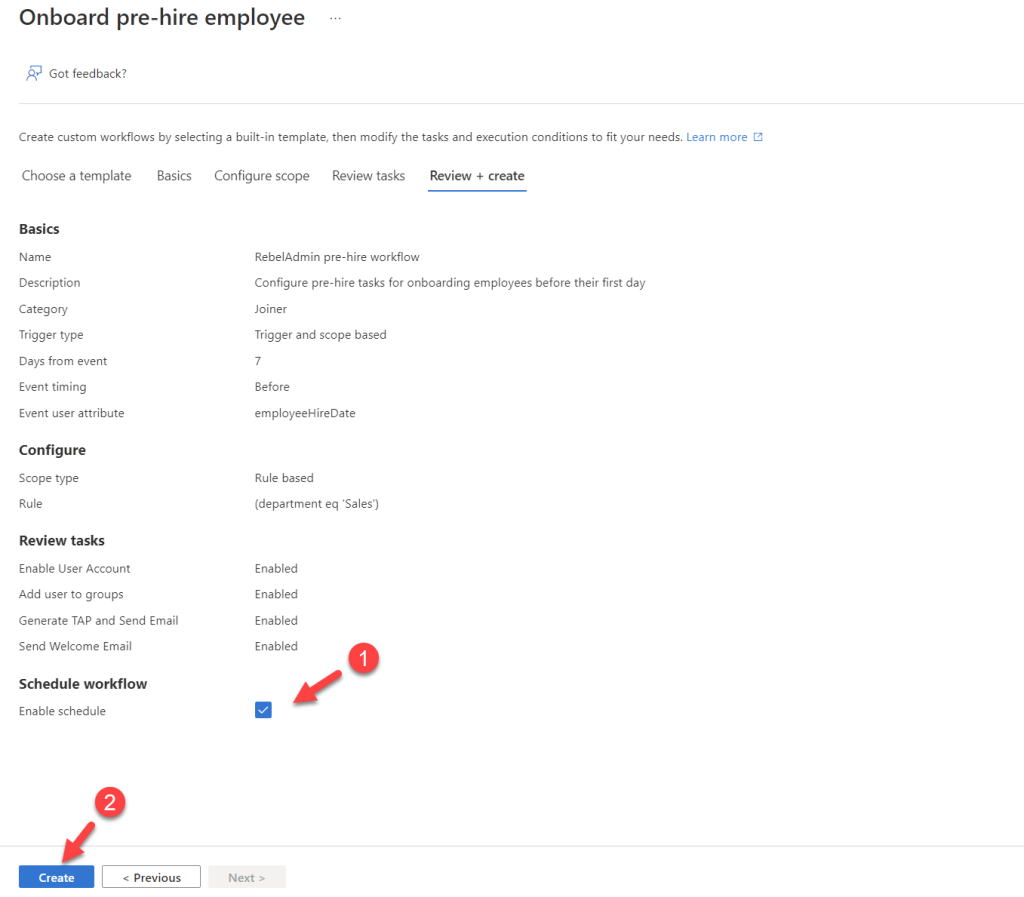This is a detailed descriptive caption for the given image:

---

The image is a screenshot from an HR software website, showing a portion of the user interface for onboarding pre-hired employees. The background is predominantly white. At the top, in bold black font, the title "Onboard Pre-Hire Employee" is displayed. Directly below, in a smaller grey font, a prompt reads, "Got Feedback?" accompanied by an icon that resembles a person with a speech bubble—depicted as a small circle above a half circle with an attached bubble. 

A thin grey line separates this header from the following instructions. Below the line, grey text explains: "Create Custom Workflows by selecting a built-in template then modify the task and execution conditions to fit your needs." A blue hyperlink labeled "Learn More" is present, suggesting additional information is available and will open in a new window or tab, indicated by a small blue box with an arrow pointing to the upper right.

Further down, navigation tabs are displayed, listing "Choose a Template," "Basics," "Configure," "Review Task," and "Review and Create," with the "Review and Create" tab being underlined to denote the current page. 

On the left side of the screen, several categories for configuration are shown: "Basics," "Configure," "Review Task," and "Schedule Workforce." Each category has a list of configurable items. A prominent blue rectangle button labeled "Create" in white font is located at the bottom of this section, next to a grey-outlined button labeled "Previous."

The image includes visual markers for guidance: a red circle numbered '2' with an arrow pointing to the "Create" button and another red circle numbered '1' pointing to a checked box under the "Schedule Workforce" category.

---